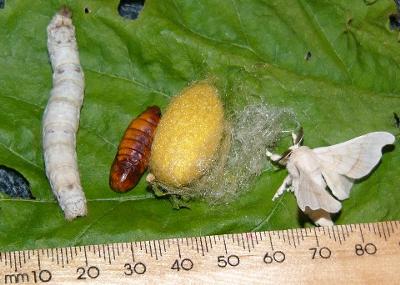The image captures the various stages of a caterpillar's life cycle meticulously arranged for scientific documentation and comparison. Set against a bright green backdrop resembling a plant leaf, the scene is centered around a wooden ruler marked in millimeters (from 20 to 80) for scale. Four distinct stages of the caterpillar are displayed from left to right. First, there's a white, elongated caterpillar. Next is a dark brown, shell-like form, presumably a transitioning stage or smaller larva. This is followed by a webby, yellowish cocoon. Finally, the sequence ends with a white form, likely an emerging moth or butterfly. The objects are positioned neatly in front of the ruler to provide clear perspective and measurement, all amidst a green background that might be a tablecloth or leaf, making the scientific purpose of the photo evident. The photo quality is noted as fairly poor, with no text other than the ruler increments visible.